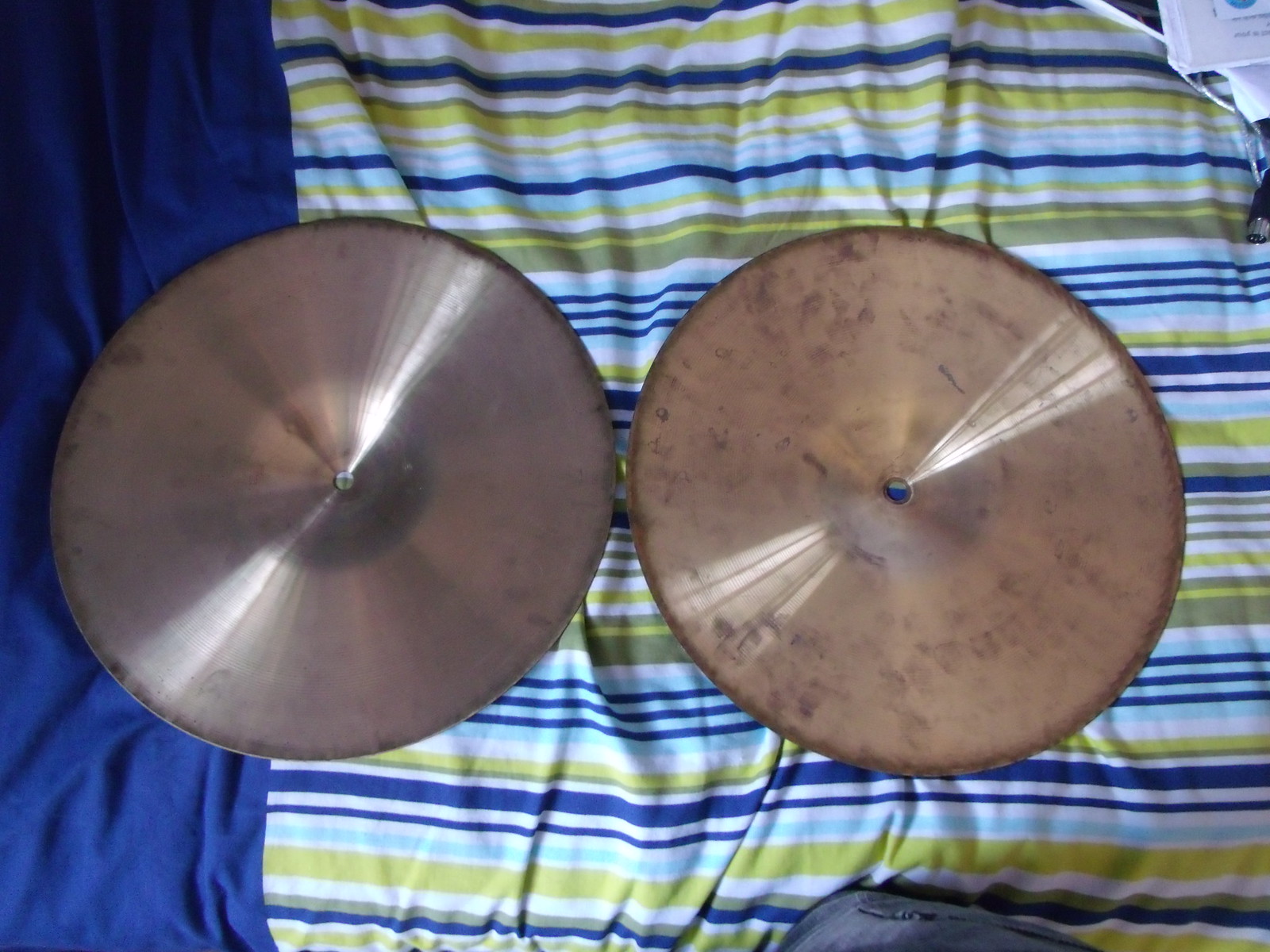This photograph captures a top-down view of a piece of fabric with distinct sections and vibrant colors. On the left side, a solid band of royal blue fabric occupies roughly an eighth of the frame. Adjacent to this, the fabric features alternating horizontal stripes in varying colors: shades of blue, yellow, white, and a patterned-blue stripe. The center of the image prominently displays two circular metal objects, possibly cymbals, resting on the fabric. These objects are distinguishable by their worn and tarnished appearance. The left disk exhibits a silver hue with noticeable black stains, scratches, and a central black screw indicative of a handle or attachment piece. Conversely, the right disk has a brownish copper tone, similarly marked with stains and a central hole, though lacking the screw or handle seen on the other. The disks' weathered conditions suggest they have been subjected to neglect or harsh elements.